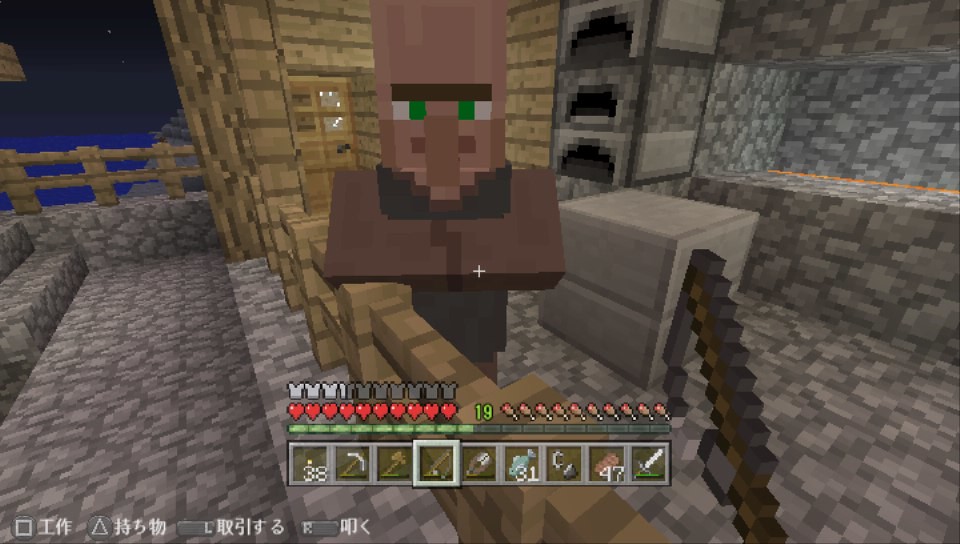The image depicts a computer-generated scene featuring a person created with blocky, geometric shapes. The character has a distinctive box-shaped head with green boxy eyes, a square purple mouth, and a vertical brown box for a nose. He is holding a brown tray, adding to the kitchen-like atmosphere. In front of the person is a wall made up of various box segments in different shades of brown, enhancing the textured background. 

Adjacent to him, there is a large gray box structure with stairs leading out of it, reinforcing the abstract and geometric style of the scene. This structure alongside two visible open-door ovens gives the impression that the setting is a kitchen, perhaps with brick ovens.

Behind the character, a tan door with windows opens out to a dark exterior, hinting at nighttime. Outside the door, there appears to be a wooden deck with a fence framing the view. In the distance, visible through the doorway, is a serene blue expanse that could be the ocean, suggesting that this beach is adjacent to the setting.